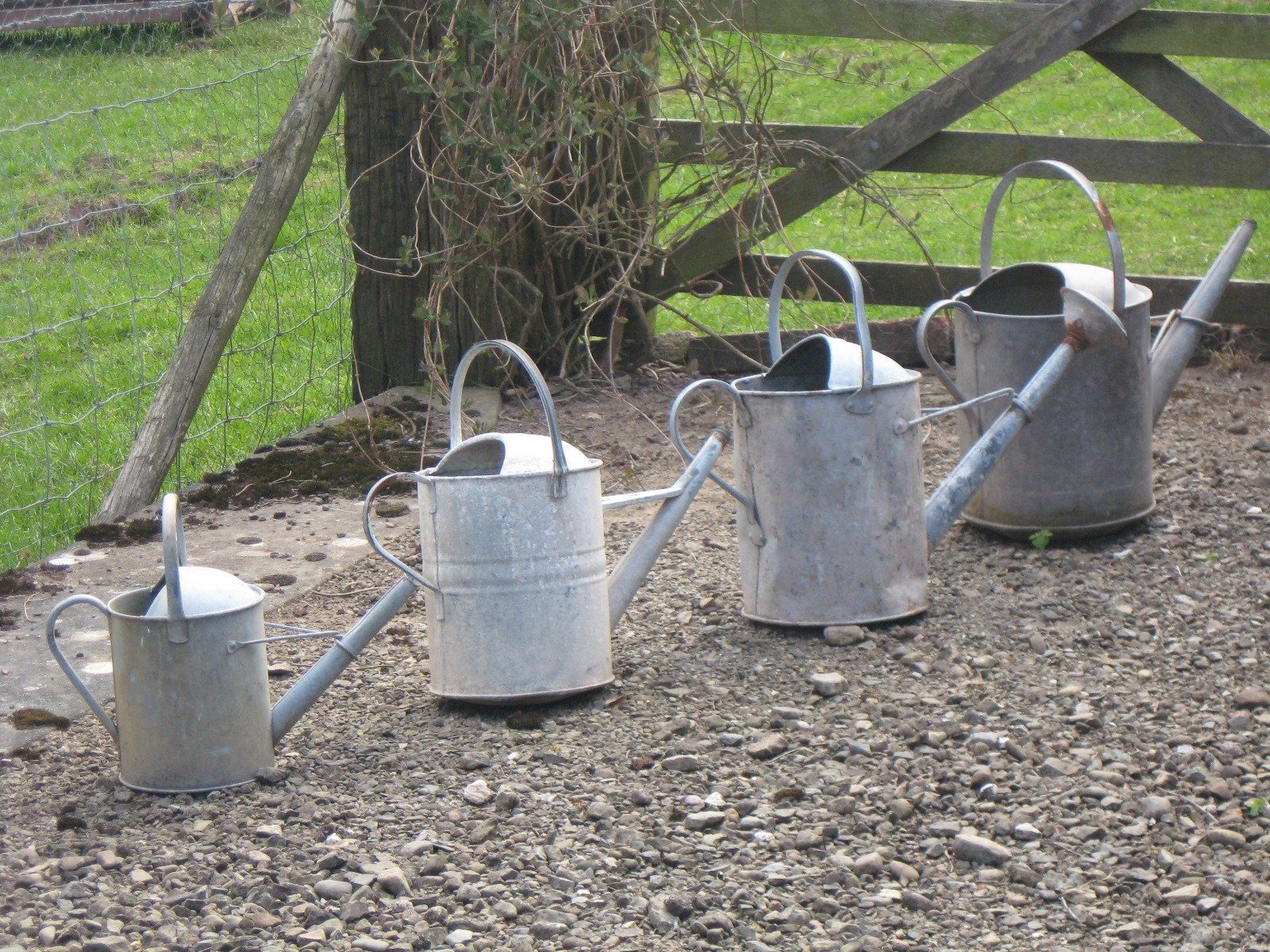The photograph captures a serene outdoor scene during a sunny daytime, centered around four tin watering cans arranged in ascending order of size, from the smallest on the bottom left to the largest on the center-right. These cans are situated within a fenced enclosure, the pen being delineated by sturdy wooden beams and cross beams supported by horizontal beams, and reinforced with wire mesh, presumably for the control of small animals. The enclosure's floor is a gravel ground comprising grey rocks with mixed shades of light and dark brown. In the background, the pen borders green grass patches interspersed with dark rut marks, possibly from animal movement. Notably, in the corner of the pen, a stump is draped with brown vines and dark green leaves. The watering cans themselves, exemplifying a cylindrical design akin to paint cans, feature a long spout emerging from the bottom, a handle on top, and another on the side. The largest can, situated near the center-right, displays noticeable rust near its spout. Overall, the composition highlights the rustic charm and functional simplicity of these garden essentials.